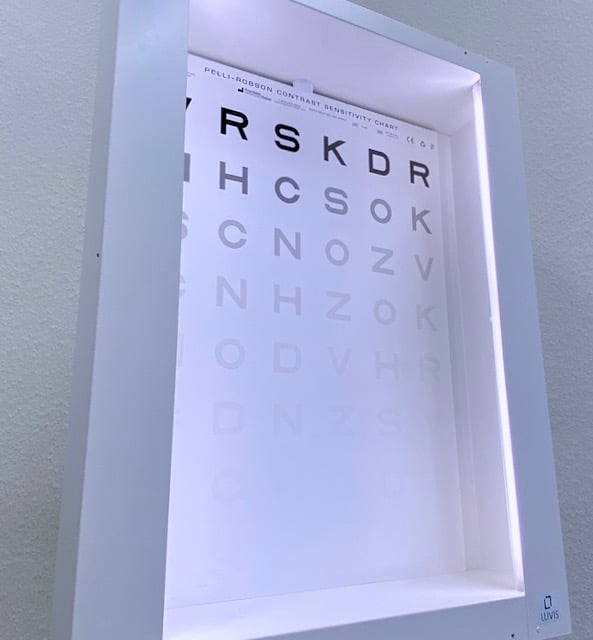This image showcases a Peli Robson Contrast Sensitivity Chart, commonly used for eye exams at a doctor's office. The chart is mounted on a white wall and is enclosed in a white frame. Small lights are embedded around the frame, illuminating the chart. In the top left corner of the chart, the letters R, S, K, D, R are clearly visible, followed by a row that includes H, C, S, O, K, among other letters. As the rows descend, the letters (C, N, O, Z, V, N, H, Z, O, K, O, D, V, H, R) become progressively harder to read, becoming particularly blurry towards the bottom. Additionally, there are smaller words under the main title "Peli Robson Contrast Sensitivity Chart," but they are not legible. The name "Louvis" appears in blue at the bottom right of the frame, though it too is somewhat blurry. A portion of the chart on the left-hand side is obscured by the frame.